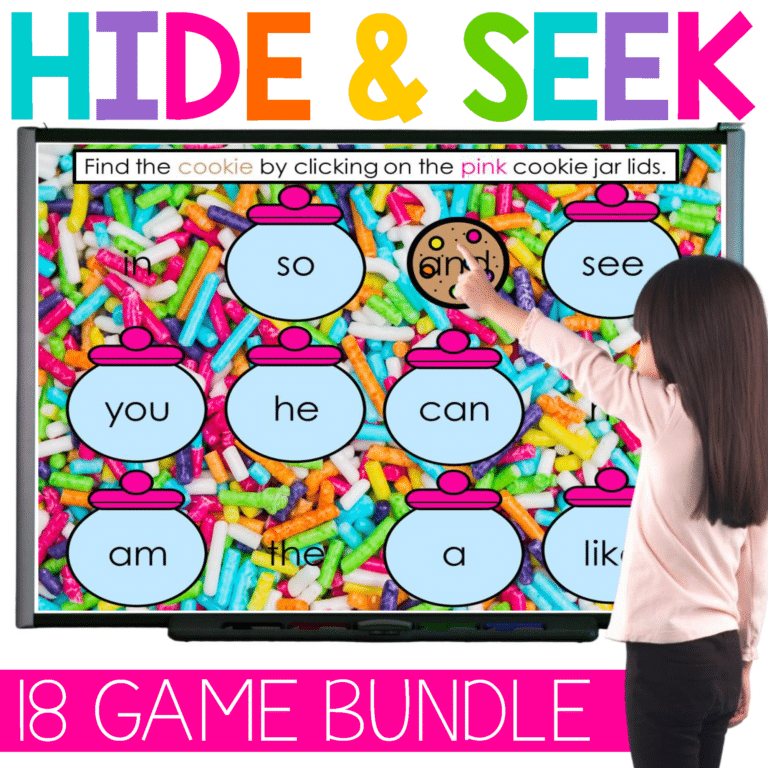The promotional image for an 18-game bundle features an engaging and colorful Hide and Seek game prominently displayed on a television screen at the center. The title "Hide and Seek" is boldly spelled out across the top in vibrant, multicolored letters: an aquamarine H, a purple I, a pink D, an orange E, a yellow N, a green S, an aquamarine E, a purple E, and a pink K. Below this flashy title, a banner on the television instructs viewers to "Find the cookie by clicking the pink cookie jar lids." The screen depicts eight cartoonish cookie jars, each with a pink lid and a light blue body, surrounded by various small, colored pieces. Positioned to the right, a small girl with long black hair, wearing black pants and a long-sleeved pink shirt, points towards a cookie labeled "and" on the screen. Although we only see her from the back, her engagement is evident. At the very bottom outside the television frame, another pink banner announces in bold white text, "18 game bundle," completing this eye-catching and interactive advertisement.